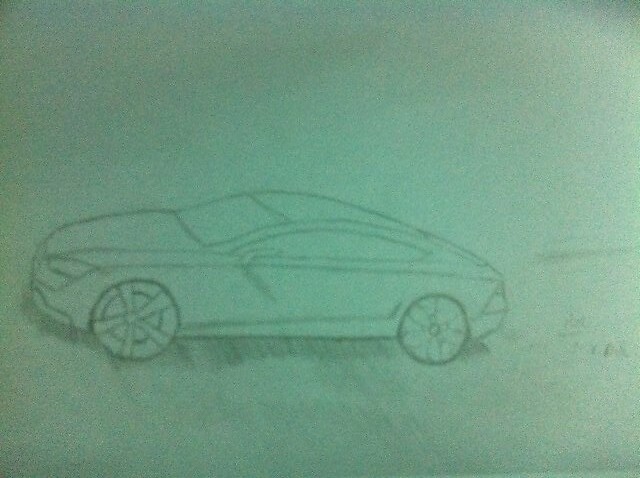The image features a pencil sketch of a two-door sports car rendered on a greenish-gray background. The car is depicted in profile, oriented to the left, revealing its sleek, streamlined design with long side windows stretching from the front to the back and a sharply slanting rear. The front hood is notably larger compared to the small trunk. The car's perspective is slightly flawed, as one wheel appears larger than the other, but both hubcaps exhibit the most intricate detailing, showcasing distinct patterns—one with a fan-like design and the other resembling petals. The sketch employs simple lines to define elements like the windshield, headlights, and rear brake lights, while the side view mirror appears misshapen. Shading beneath the car, achieved through diagonal pencil lines, adds dimension but lacks precision, suggesting an uncertain grasp of light and shadow. The overall drawing is rudimentary, emphasizing the car’s form more than precise detail.